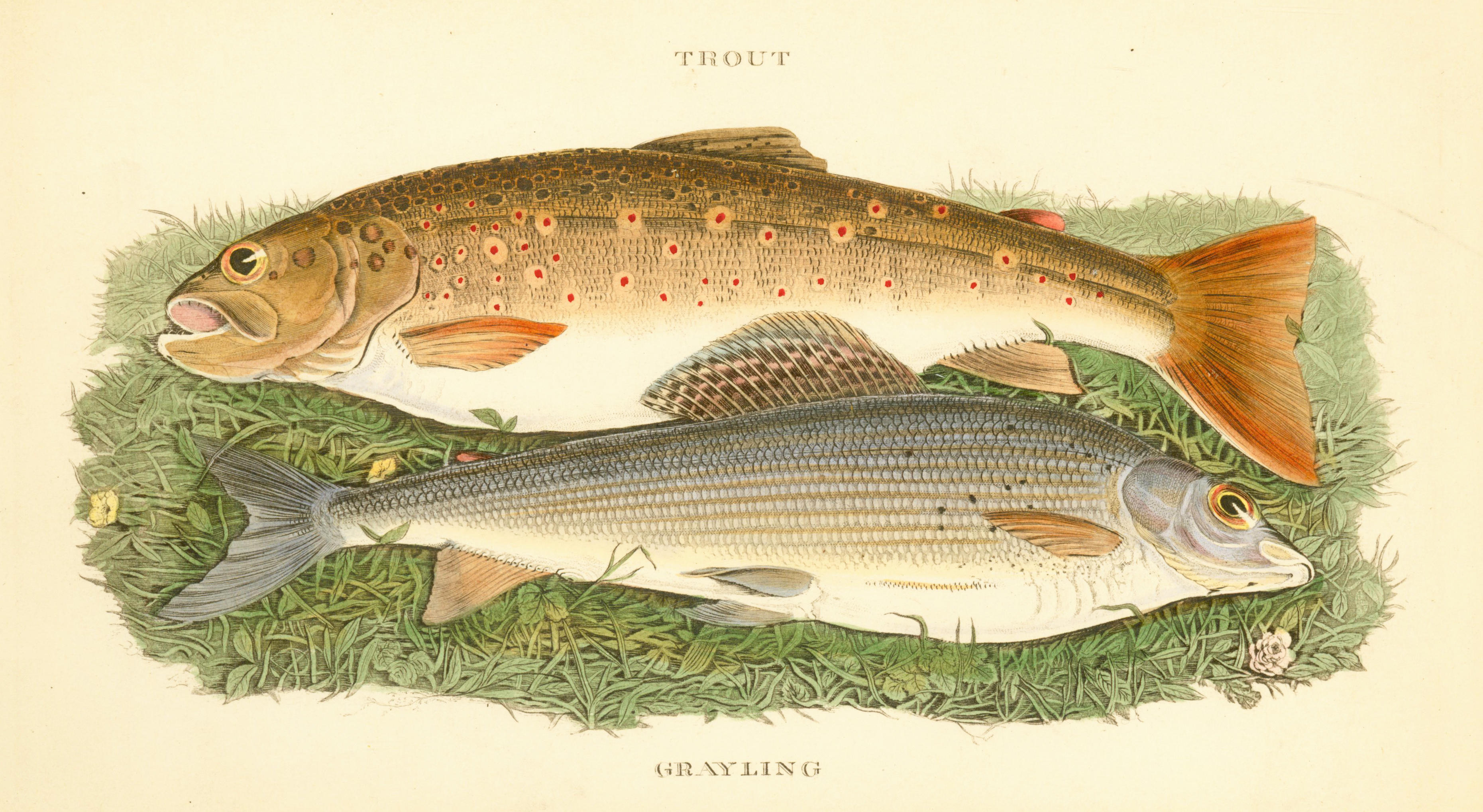The image depicts a detailed illustration from a book, showing two fish laid out on a rectangular patch of green grass against a yellow background. Both fish are positioned on their sides, with one facing left and the other facing right. The top fish, labelled "trout," is a brownish-orange color with light green hints and red-speckled spots. Its mouth is open, and it appears to be staring off into the distance. The bottom fish, labelled "grayling," has a silvery-gray body with tight scales and light brown fins. It has a closed mouth and similarly stares off into the distance. Both fish share a similar eye color, a light golden or brown shade, and the entire illustration is rendered in a landscape aspect ratio, suggesting it is from a textbook or a fancy print.